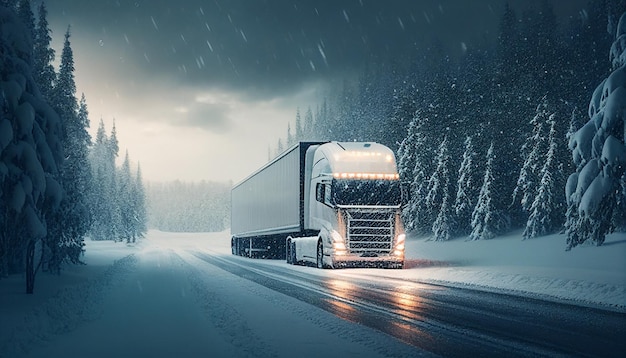The image showcases a serene yet cold atmosphere, with a large white semi-truck traveling on a snow-covered road, illuminated by its bright headlights. Captured from the front, the truck appears in motion, evidenced by light trails and snowflakes frozen mid-fall. Flanking the road are towering trees heavily laden with snow, suggesting recent or ongoing snowfall. The overcast, gray sky enhances the chilly and dim ambiance of the scene, with the dark tones of the environment contrasting sharply with the truck's lights. The setting is decently lit, hinting at either early evening or dusk. The overall clarity and quality of the image suggest it could be a highly realistic, perhaps AI-generated graphic. The wet, snowy road and plentiful snow on the ground emphasize the wintry conditions, creating a vivid, detailed depiction of a snowy night journey.